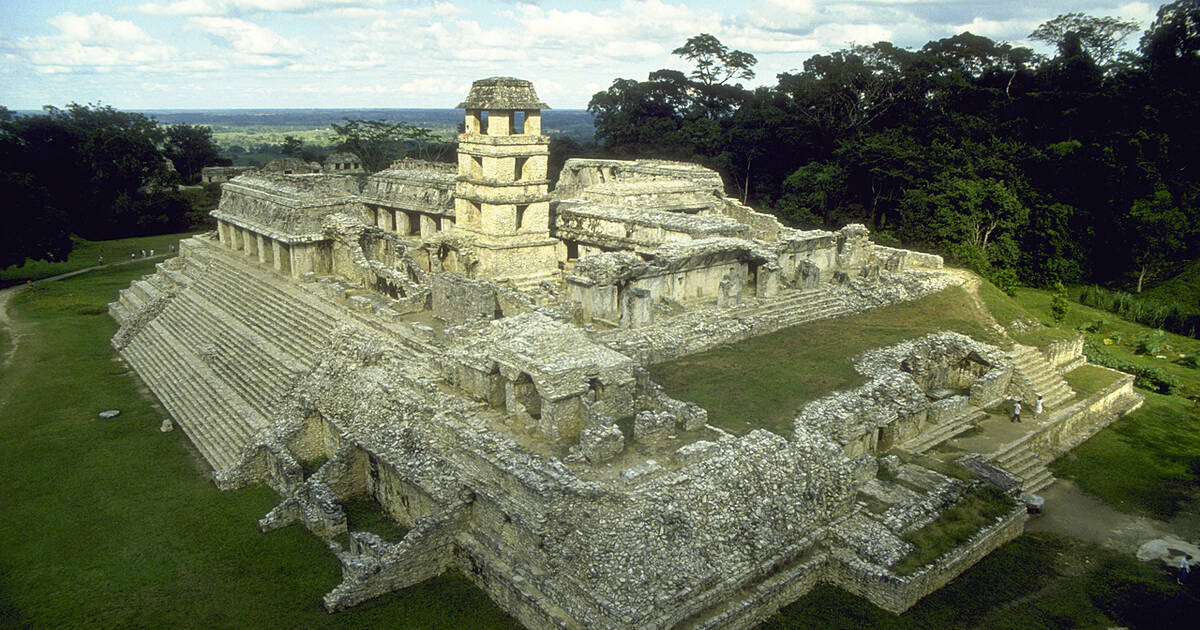The photograph showcases impressive ancient ruins nestled in a grassy expanse, likely a former imposing structure now in decay. Dominating the scene are three flights of wide, imposing stone stairs leading up to a central tower, which stands around three to four stories tall, punctuated with windows. The ruins, composed of simple gray stone, are surrounded by a blend of tall, bushy trees and open grasslands, indicating a rich history despite its weathered state. Details suggest potential historical significance, possibly as meeting halls or religious structures. Noteworthy is the presence of three tiny human figures; two are ascending the stairs, and one appears to be walking away, emphasizing the grand scale of the ruins. The photograph's day setting includes a blue, cloud-dotted sky, adding to the serene yet historic ambiance of the site.